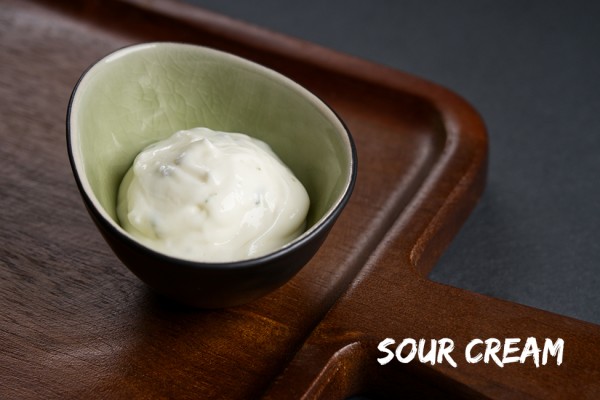The image is a color photograph featuring a close-up of a pewter dish with an artistic shape, slightly elevated on one side, containing a dollop of thick white sour cream. The interior of the bowl has a matcha green ceramic finish, contrasting with its black or dark brown exterior. The bowl is positioned slightly to the left on what appears to be a heavy, dark wooden tray or cutting board, which rests on an even darker countertop. The deep wooden board is designed to catch any drippings, hinting at its utilitarian purpose in a kitchen or cooking scenario. The background and foreground colors create a dramatic, dark setting that highlights the brightness of the sour cream. A large white text in the lower right corner of the image reads "SOUR CREAM," clearly identifying the dish's contents. This composition focuses entirely on the sour cream, inviting the viewer to imagine it as an essential ingredient awaiting the perfect dish.